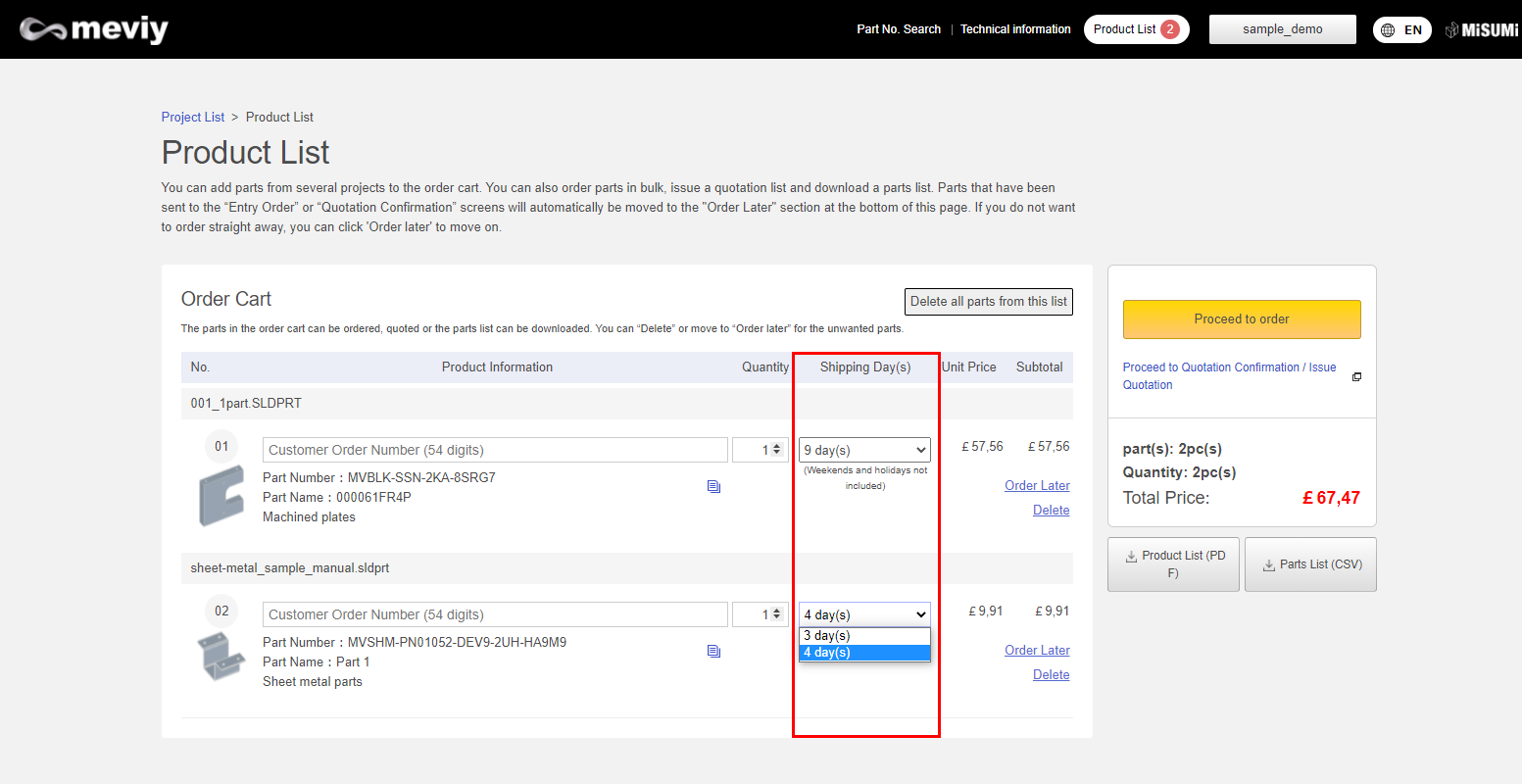The screenshot depicts a purchasing program called MEVIY, identified by its black ribbon at the top and a product emblem featuring a white infinity symbol. The platform appears to be European-based, as indicated by the use of the Euro currency. The product list includes two items, both of which seem to be metal parts specified by customer order digits. The first item resembles a metal 'C' shape, akin to what one might expect a toddler's letter 'C' to look like. The second item looks like an anchor designed to support an object against the bottom of a desk or ceiling.

Shipping details for the first product indicate a delivery time of nine days, while the second product has a drop-down menu showing options for either three or four days. An orange-yellow "Proceed to Order" button is positioned to the right, followed by a summary indicating the order consists of two pieces of each product. The total price for the order is listed as €67.47.